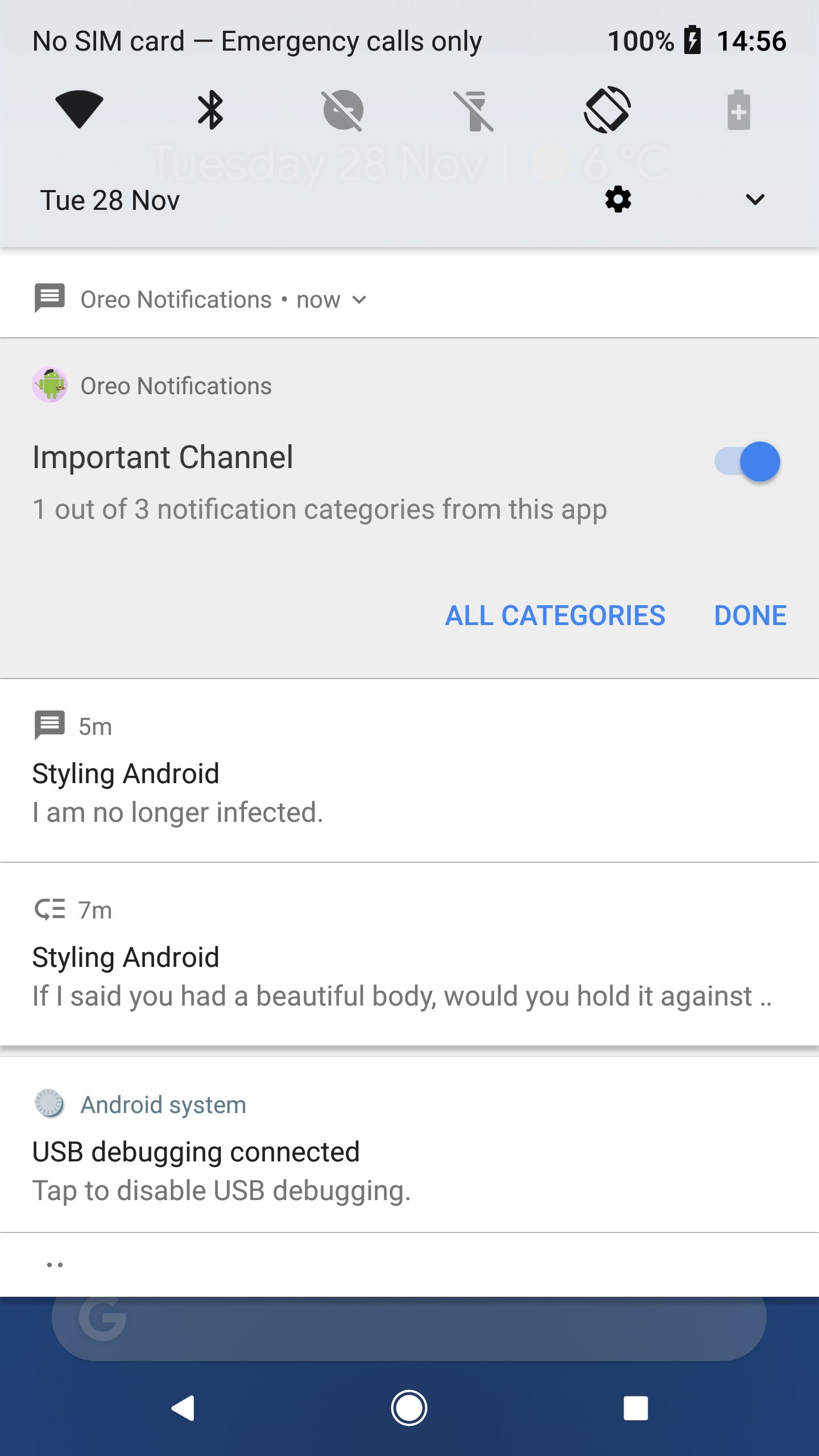This is a detailed screenshot from an Android smartphone's home screen, capturing a segment of the user's notifications and system status. 

At the top of the screen, a light blue status bar displays "No SIM card," indicating that only emergency calls are possible. The battery is fully charged at 100%, and the time is 14:56. Various status icons follow this information. Below the status bar, the date "Tuesday, 28 November" is displayed along with additional icons.

Beneath this upper section, there is a prominent gray notification box titled "Oreo notifications." It details an "important channel," which is one out of three notification categories from a specific app. The box includes a small blue circle icon with a light blue bar extending from its left side. In the bottom right of this notification box are the options "All categories" and "Done," highlighted in blue.

The subsequent notifications are detailed as follows:
- A notification with a symbol indicating "5M, styling Android" and the message "I am no longer infected."
- Another notification marked with a different symbol indicating "7M, styling Android" and the partial message "If I said you had a beautiful body, would you hold it against..."
- An Android System notification with a symbol indicating "USB debugging connected, tap to disable USB debugging."

At the very bottom of the screen, there's a dark blue horizontal rectangle containing the Google search icon ("G") and a search bar. The navigation bar at the absolute bottom comprises three standard Android navigation buttons: a white triangle pointing left (Back) on the left, a white circle (Home) in the center, and a white square (Recent Apps) on the right.